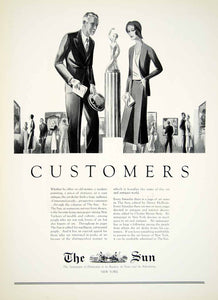The black-and-white newspaper page features a detailed illustration at the top half, occupying almost half the page. This vintage-style illustration depicts an art gallery scene with multiple figures in the background viewing framed artwork on the walls. Dominating the center of the illustration stands a tall pedestal holding a statue—reminiscent of a trophy—with a figure raising its arm in triumph. To the left of the statue, an older man with whitish hair, clad in a dark suit and tie, holds a paper in his right hand and a top hat in his left. Opposite him, to the right of the statue, a woman dressed in a long skirt, light-colored shirt, blazer, and hat stands holding a pocketbook. Both figures are absorbed in looking up at the statue. Below the illustration, the large, bold headline "Customers" is printed, followed by two paragraphs of text in two columns, too small to decipher. At the very bottom of the page, in decorative gothic typeface, are the words "The Sun" with an image inscribed between 'The' and 'Sun'. A bold black line marks the end of the page.